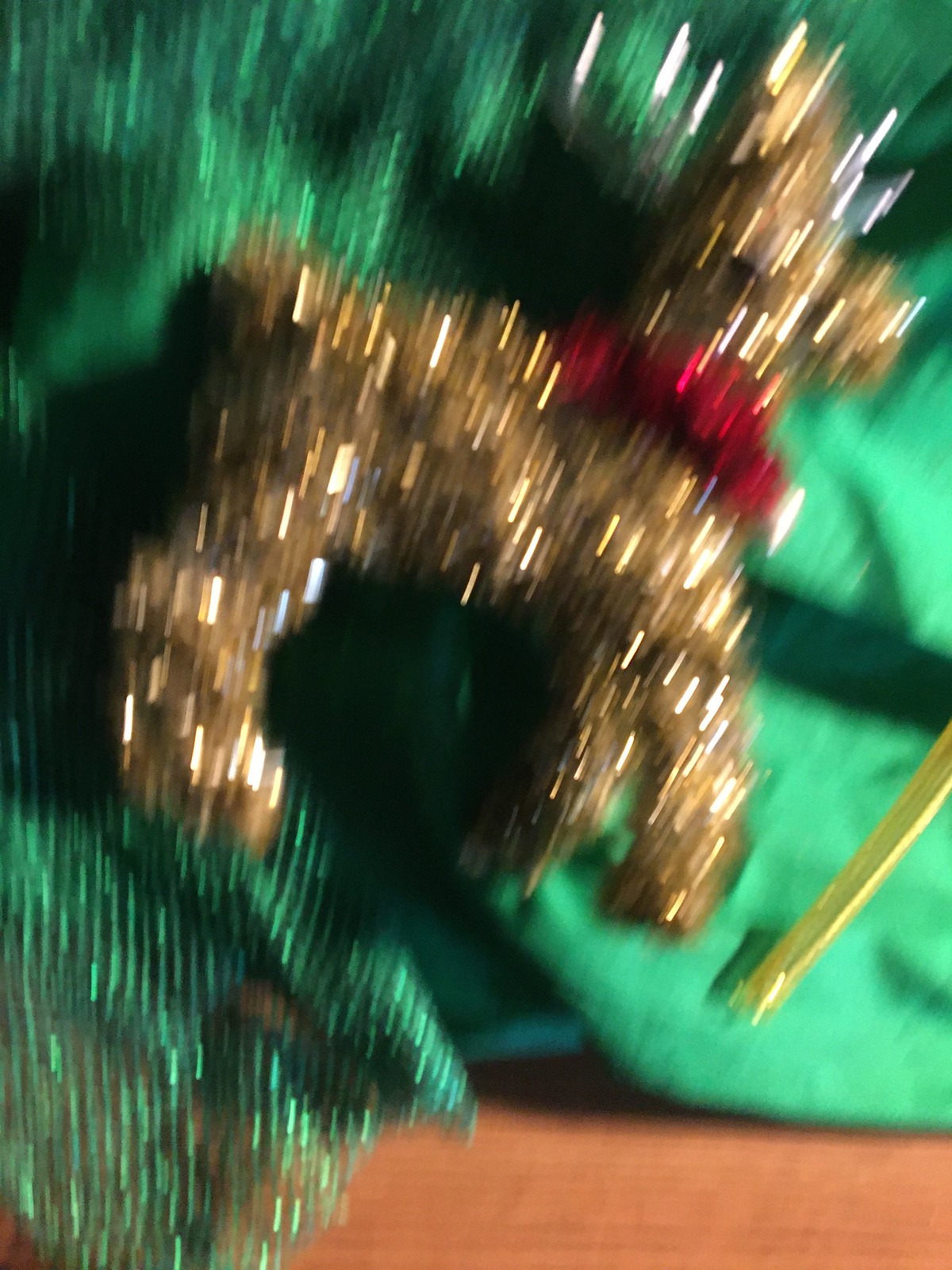This image, though blurred, appears to depict a festive holiday scene featuring a reindeer ornament suspended on a Christmas tree. The reindeer ornament is brownish gold in color and adorned with a striking red scarf around its neck. The green background suggests the boughs of the Christmas tree, while the presence of a visible wood floor indicates that the ornament is hanging near the bottom of the tree. The overall ambiance evokes the warmth and charm of holiday decorations, capturing a small but endearing detail of a festive setting.